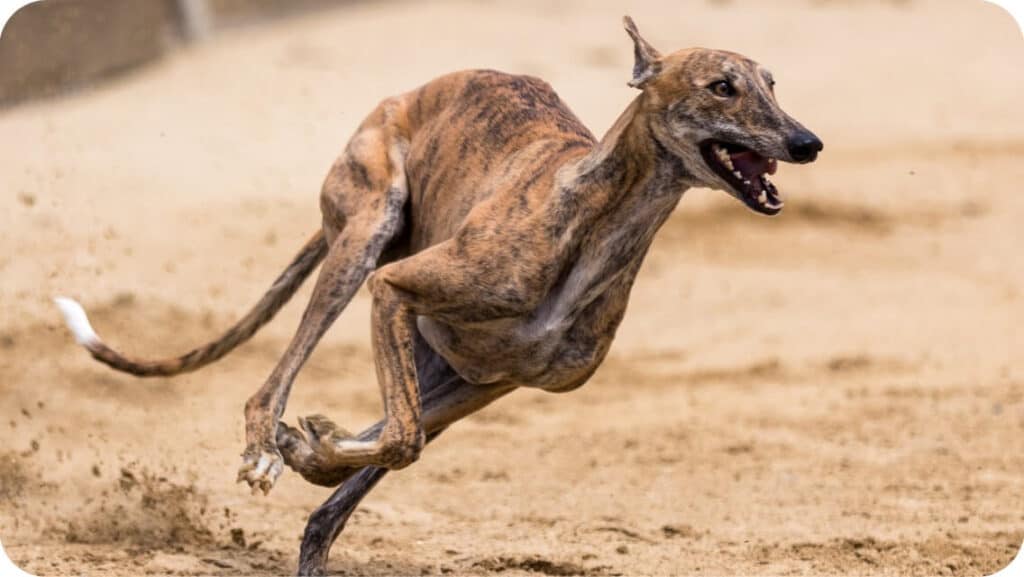The photograph captures a wiry greyhound in full motion, racing across a sandy track, its sleek, slender body and long legs indicating the athletic prowess typical of its breed. The greyhound's coat is primarily light brown, interspersed with dark brown, almost black spots, and accented with touches of white on its undercarriage, the tips of its feet, around its jawline, and at the tip of its long tail. The dog’s mouth is open, revealing pointy teeth, and one of its triangular ears is perked up as it faces towards the camera and to the right, with its long snout leading the way. The background of the image is mostly a blur of beige sand kicked up by its powerful stride, emphasizing the speed and intensity of the race. Although this appears to be a race, the greyhound lacks any identifying markers such as a racing number or collar, focusing all attention on the dog's grace and agility.